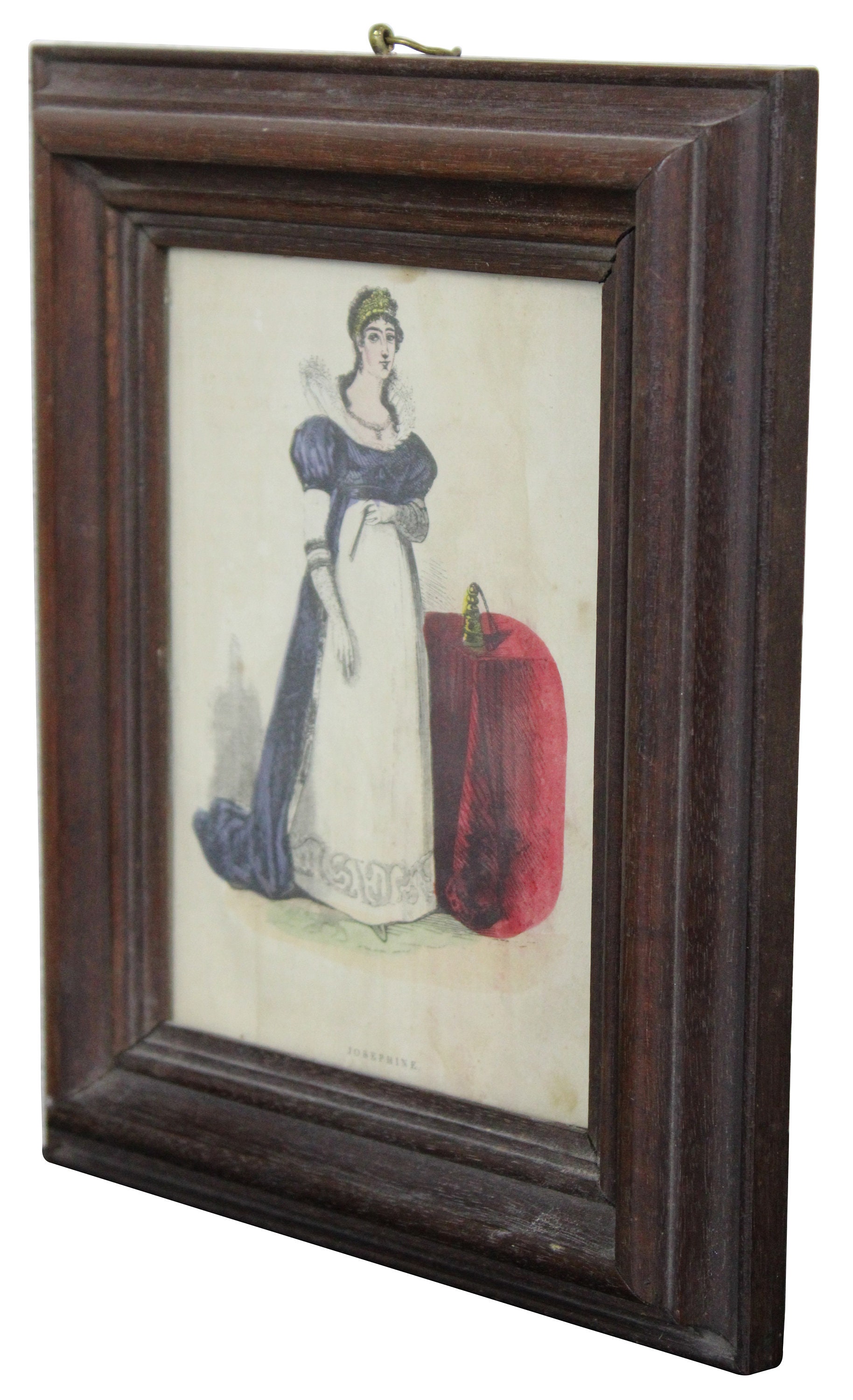This is an image of an old-fashioned, hand-drawn artwork framed in a very thick, dark wood frame, lined with curves and some scuff marks, giving it an antique feel. The painting, possibly from the 1500s or 1600s, is small and shows signs of age with fading paint and minor scratches. It features a noblewoman in a detailed white and blue dress with black puffy sleeves and a trailing train. Her hair, which is brown and ends in a braid, appears to be adorned with a golden crown. The woman stands confidently next to a table draped in a vibrant red cloth, on which rests a golden object, possibly a cone, along with another indistinct green item. The background of the artwork is stark white, with a shadow cast behind the figure, and there is a signature at the bottom that is not legible from the current view. This painting, with its meticulously captured details and aged frame, looks like a collectible piece one might find on an antique marketplace.